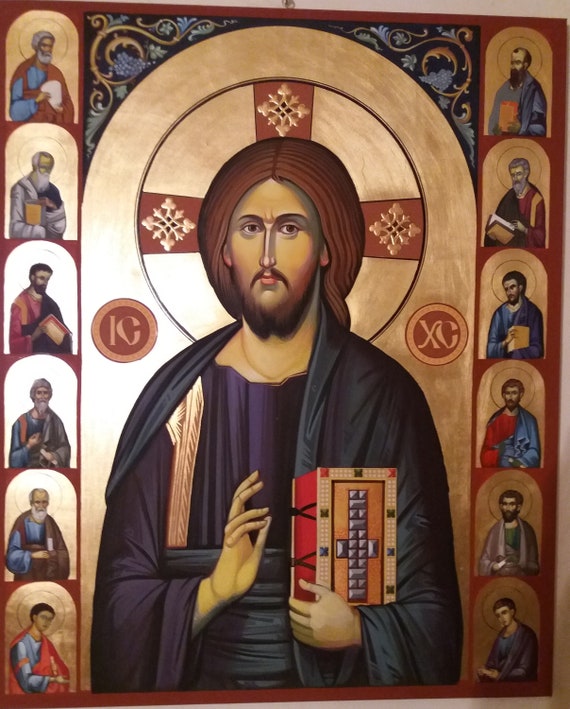This is a highly detailed medieval-style religious painting of Jesus Christ, who is depicted centrally before a grand arch with a golden halo featuring a cross behind his head. Jesus, with long brunette hair and a serious demeanor, is adorned in a purple robe and a navy blue overcloak. In his left hand, he holds a decorated box, which appears to be a Bible embellished with gemstones and a silver-studded cross, featuring red pages and a black binding. His right hand is raised in a prayer sign. Surrounding Jesus are 12 apostles, each situated in small inset circles along the frame, attired in variously colored robes. These figures are depicted in different gestures, some holding books and others with hands in prayer. Accompanying the scene is intricate detailing, including a swirl motif with grapes at the top. The gold metallic background enhances the sacred ambiance. The letters "IC" and "XC" are prominently placed on either side of Jesus, emphasizing the holy context.